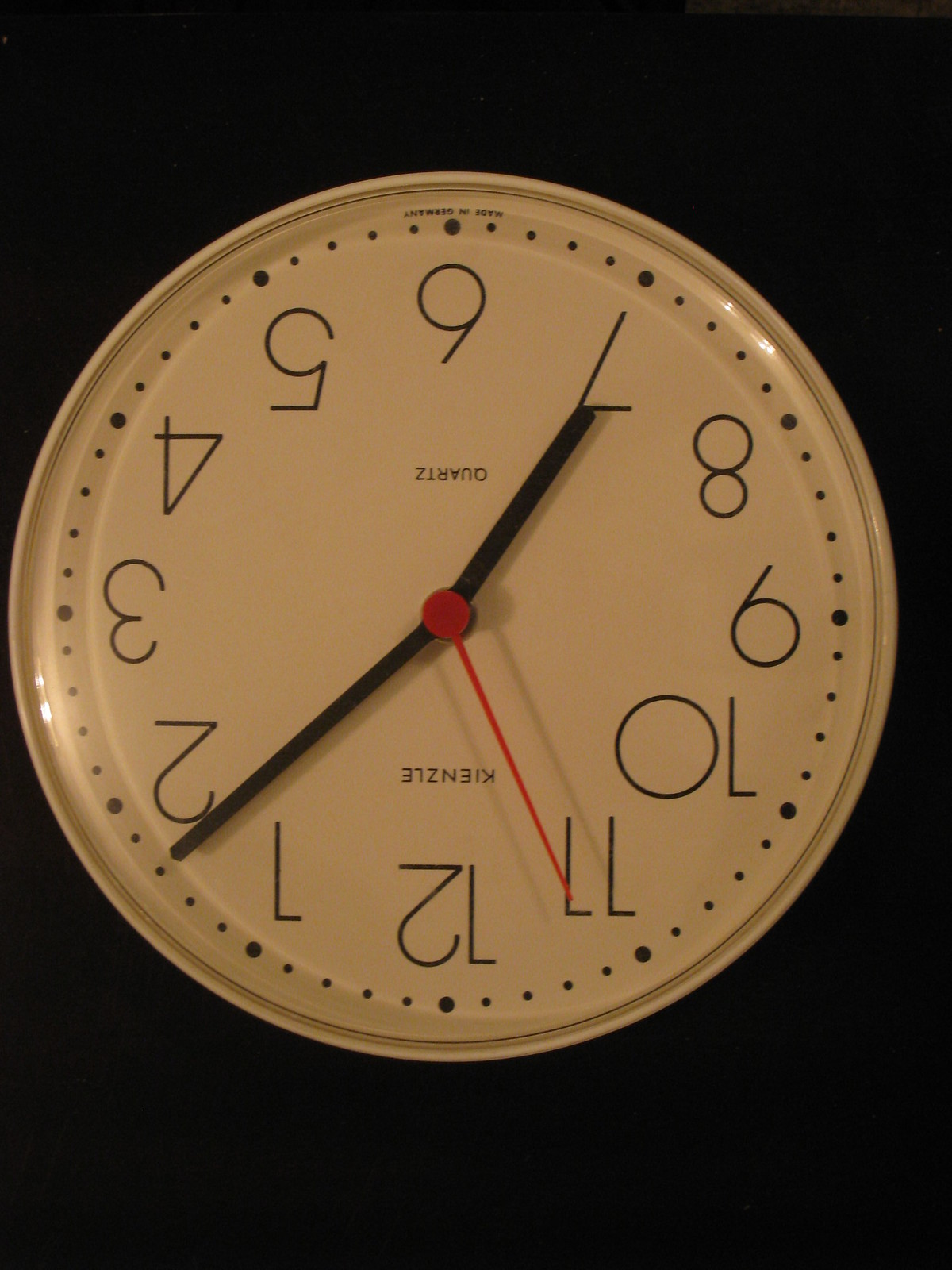The image features an upside-down white clock set against a plain black background. The clock face displays the numbers 1 through 12 and is marked by fine tick marks. The shorthand rests on the 7, while the longhand lies between the 1 and 2, indicating a time of approximately 7:08. A slender red second hand, with a round section at its base, is stopped at 57 seconds. Under the 12, the letters "K-I-E-N-V-L-E" are inscribed, and above the 6, the word "corpse" is written. Shadows cast by the clock hands are visible, adding subtle depth to the image.